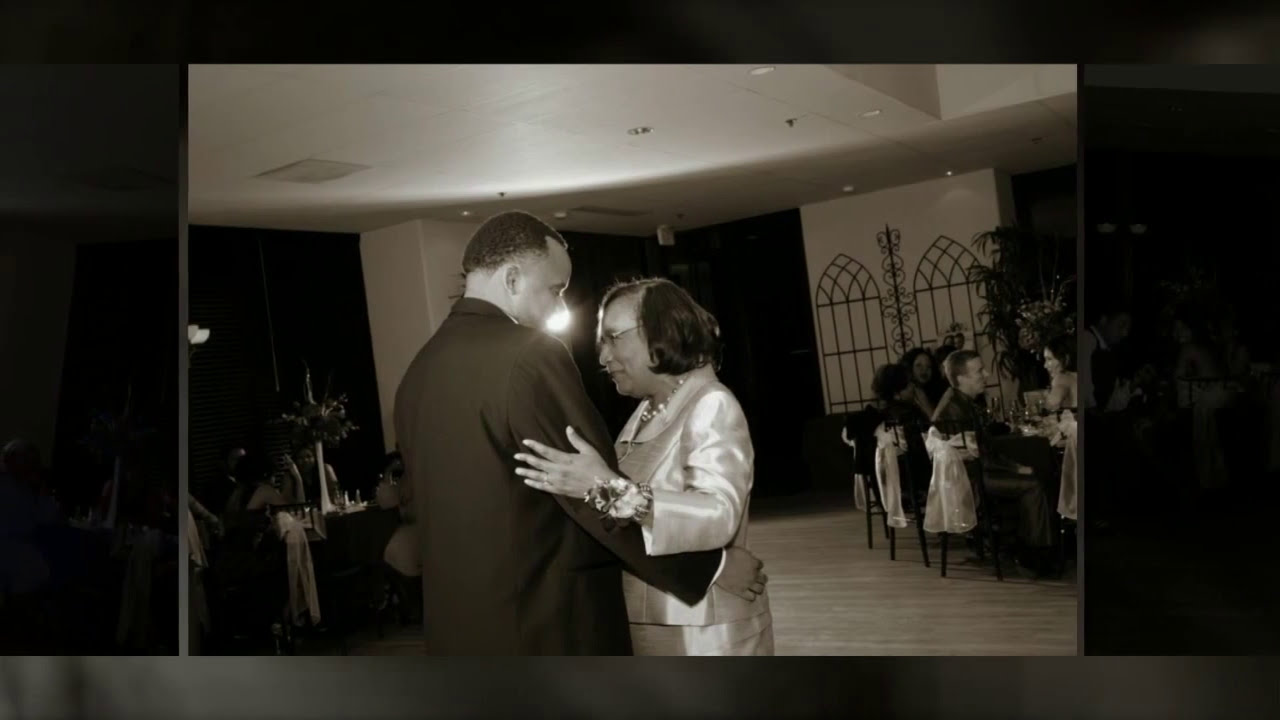In this evocative black-and-white photograph, a touching moment unfolds as a younger man, dressed in a dark suit with cropped hair, gently dances with an elderly woman in a light-colored, silky suit. She's adorned with a corsage on her left wrist and wears glasses, her short, dark hair styled neatly. Their tender slow dance takes place in the center of a spacious, elegant room with a light wooden floor, suggesting a formal event such as a wedding or perhaps an anniversary celebration. Seated at round tables in the background, a diverse group of attendees enjoys dinner and drinks, adding to the scene's atmosphere of joyous togetherness. The photograph, framed with a gray metallic border and footer, captures the essence of a special dance, hinting at a close relationship, possibly between mother and son or a long-married couple, under the soft illumination that accentuates their connection.